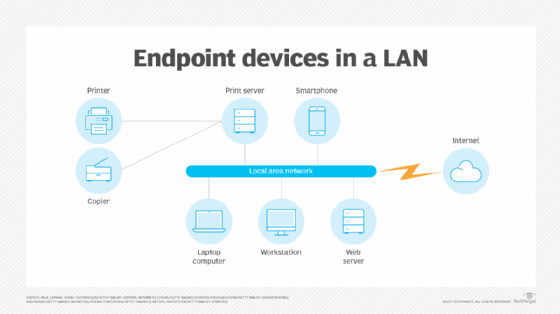The illustrated image depicts endpoint devices in a LAN (Local Area Network) on a white background framed by a light grey border. At the top, in black font, it reads "Endpoint Devices in a LAN." The diagram visualizes the connections within a network, starting with three light blue circles on the far left labeled "Printer" and "Copier." Both of these devices are connected via black lines to a central "Print Server," which in turn connects downward to a blue oval labeled "Local Area Network." From the right side of the blue oval, a line leads to a "Smartphone," while underneath, three more devices are connected: "Laptop Computer," "Workstation," and "Web Server." Each device is represented by a small cartoon icon. Additionally, a lightning bolt symbol emanates from the local area network, leading to a final circle labeled "Internet," illustrated with a cloud icon.